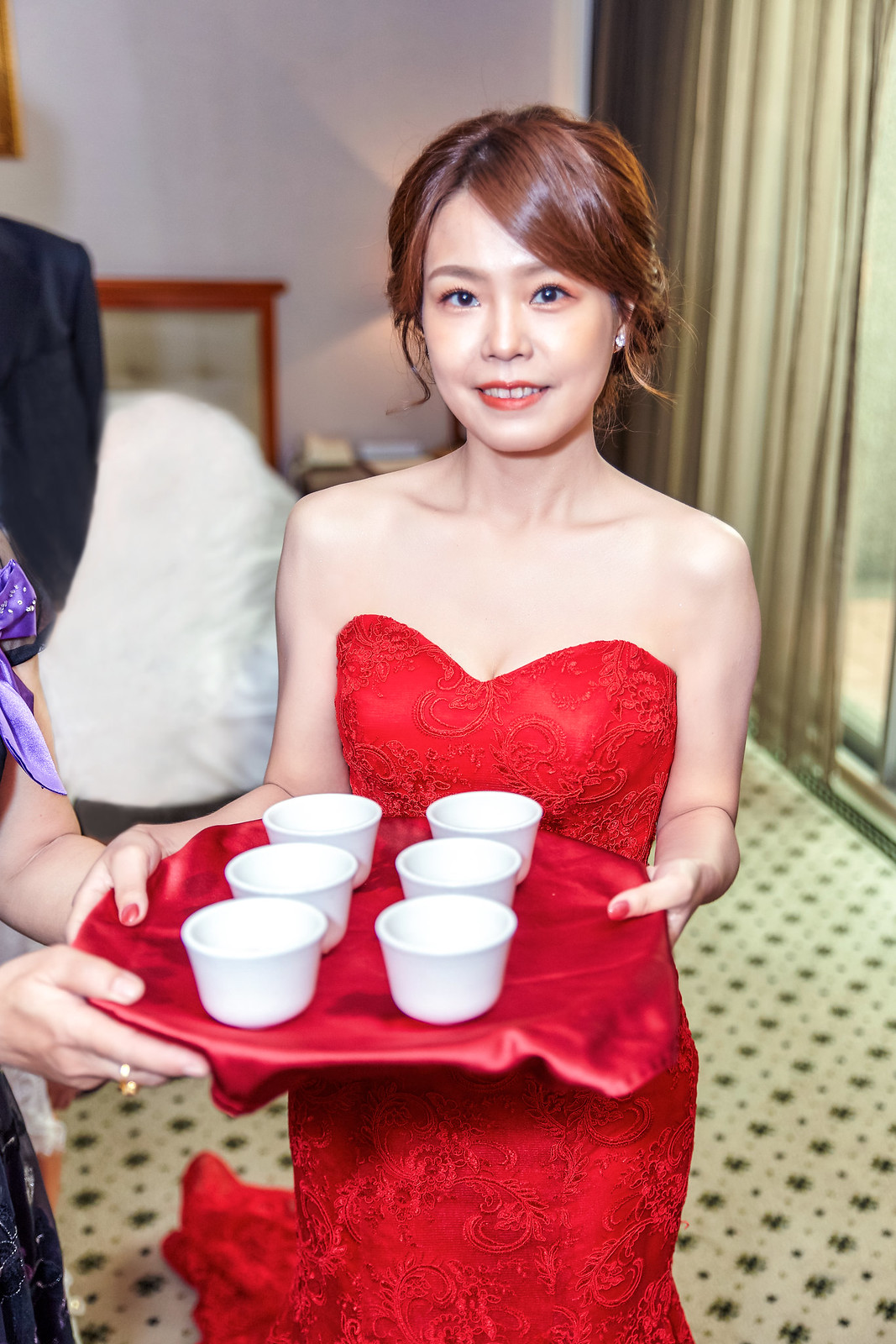The image features an elegant Asian woman with light brown hair styled in an updo, accented by side-swept bangs. She has pale skin, dark eyes, and wears subtle eye makeup with red lipstick, highlighting her bright smile. Clad in a vibrant, strapless red ball gown featuring a raised floral pattern, she exudes sophistication. Her nails are painted pink. The woman is holding a tray draped in red satin, on which six white cups are arranged in two vertical rows of three. Assisting her from the left, another woman's hand is visible, adorned with a golden ring and part of a purple bow on her dress. The background reveals a light-colored, patterned floor with black symbols, a sliding glass door covered by sheer beige curtains on the right, and a glimpse of a bed with white sheets and a cushioned, warm chestnut brown frame on the left.